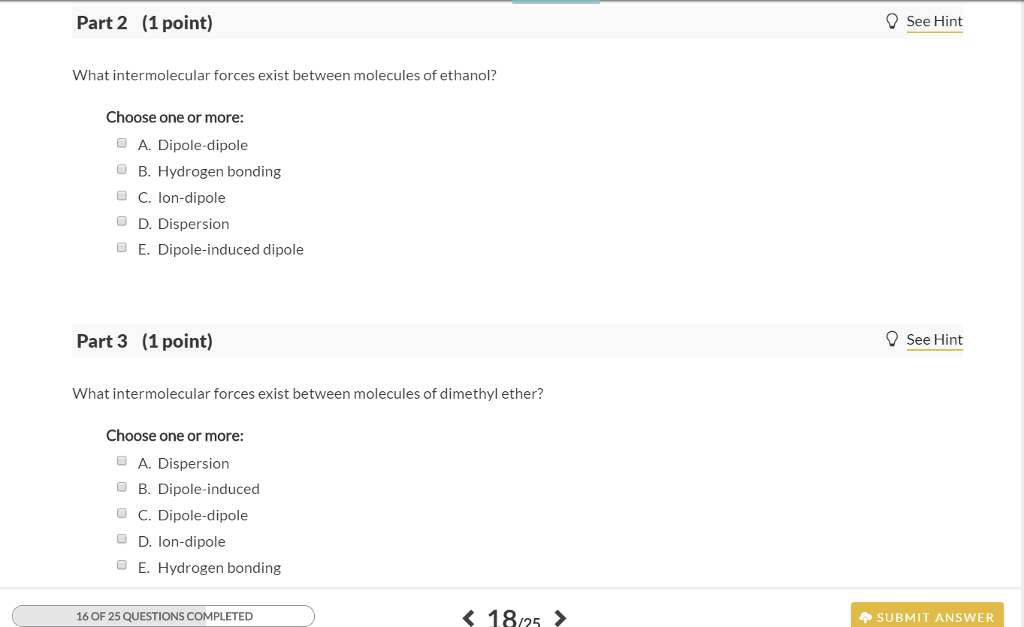**Detailed Screenshot Description:**

The screenshot captures a digital test interface, seemingly part of an online workbook or educational website, containing multiple-choice questions related to chemistry. The layout is user-friendly with clearly distinguished sections.

At the top of the screenshot, a gray background with a thin dividing line demarcates the header. In bold black letters, it reads "Part Two (1 point)," indicating the section and points allocated. Adjacent to this, on the right-hand side, there's an icon resembling a light bulb accompanied by the text "See Hint," underlined in yellow, suggesting it is a clickable element that provides additional information or clues.

The first question presented asks: "What intermolecular forces exist between molecules of ethanol? Choose one or more." Five possible answers are listed:
- A. Dipole-dipole
- B. Hydrogen bonding
- C. Ion-dipole
- D. Dispersion
- E. Dipole-induced dipole

None of the options have been selected, indicating the test-taker has not yet answered.

Below this, the next section begins with a header similar to the first: "Part Three (1 point)." To the right, the “See Hint” option is available again. The second question reads: "What intermolecular forces exist between molecules of dimethyl ether? Choose one or more." The possible answers, which mirror those of the previous question, are:
- A. Dispersion
- B. Dipole-induced dipole
- C. Dipole-dipole
- D. Ion-dipole
- E. Hydrogen bonding

At the bottom of the screenshot, a shaded area (about two-thirds covered) indicates progress with the text "16 of 25 questions completed." There is a counter "18/25" flanked by navigation arrows, and a prominent "Submit Answer" button highlighted in yellow, suggesting the user can submit their responses.

Overall, the screenshot offers a comprehensive view of the testing interface, including question prompts, answer options, progress tracking, and interactive elements for additional hints.